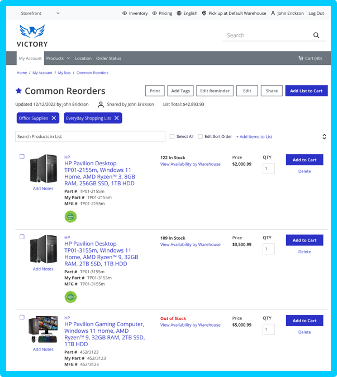The image depicts an ordering page from a company named "Victory," identifiable by the "Victory" text at the top left, accompanied by an eagle logo. The header of the page includes a navigation bar with various clickable options and a search bar on the right side. 

Below the header, the page title "Common Reorders" suggests that it is a section for frequently reordered items. The section includes sorting options such as price and other categories, though some of the text in clickable squares is illegible. 

The main content showcases three items, which appear to be computer towers, specifically HP Power Desktops. Each item listing includes a detailed product description, the price, quantity selection, and an "Add to Cart" button. The entire page is outlined in blue, providing a clean and organized interface for users.